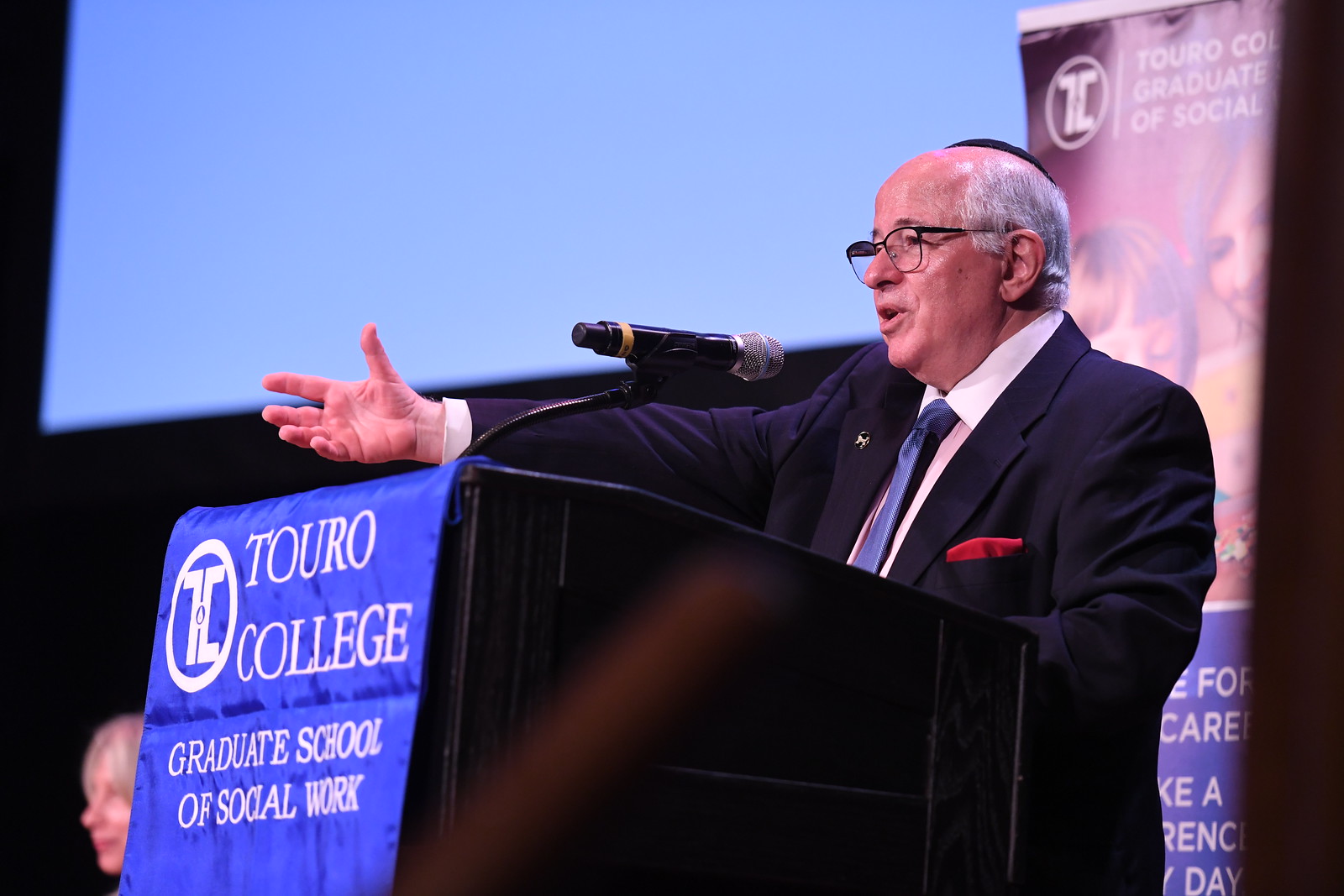This image captures a wide rectangular view of a man standing at a podium, which is positioned at the bottom of the frame. The man, who has pinkish white skin and is balding with white or gray hair, is facing somewhat to the left in a diagonal stance. He is dressed in a blue suit that resembles a sports coat, complemented by a white collared shirt, a blue metallic tie, and a red pocket square or handkerchief. He wears eyeglasses and is in the middle of speaking, with his left arm extended horizontally and a microphone in front of him emerging from the podium.

The podium itself is black and prominently features a bright blue banner with white embroidered text reading, "Turo College Graduate School of Social Work." A white circle logo containing the letters "T" and "L" is located to the left of the text. The background of the image is predominantly blue, possibly from a blank screen set up for a presentation. Additional banners are visible but partially obscured behind the speaker, indicating the same affiliation with Turo College.